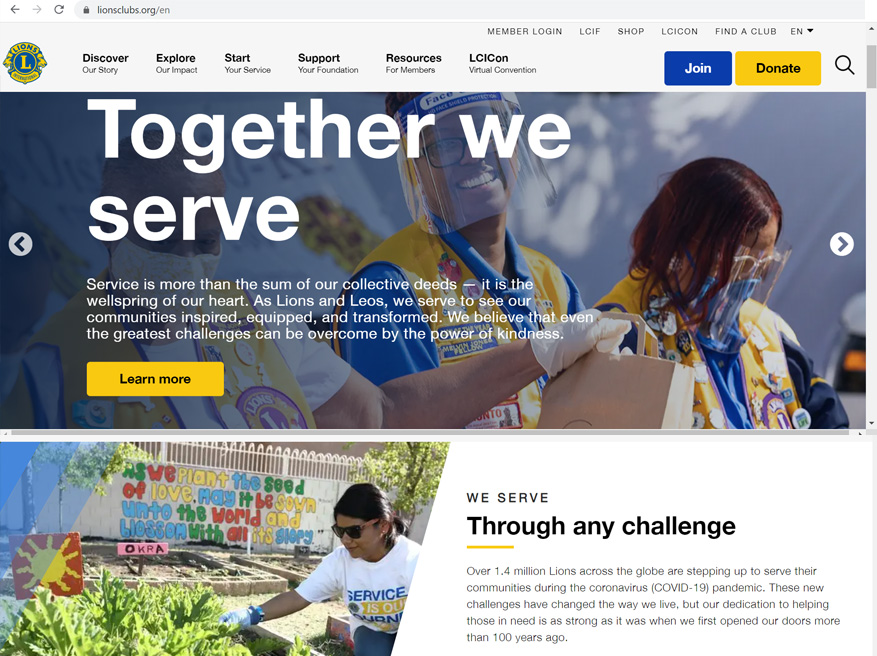This image is a screenshot of the English version of the Lions Club International website, found at lionsclub.org. 

In the upper left corner of the webpage, the Lions Club logo is prominently displayed. The logo resembles a crest with a large 'L' in the center, and it is designed in blue and yellow colors. 

At the top of the webpage, there is a navigation bar with several links for easy browsing: 
1. "Discover Our Story"
2. "Explore Our Impact"
3. "Start Your Service"
4. "Support Your Foundation"
5. "Resources for Members"
6. "LCICON, Virtual Convention"

To the right of these links are two prominent buttons: a blue one labeled "Join" and a yellow one labeled "Donate." Additionally, there is a magnifying glass icon for search functionality.

The main body of the webpage is dominated by a large banner featuring a vivid image of Lions Club members packing brown paper bags of food and distributing them to those in need. The banner carries the title "Together We Serve" and includes a brief description emphasizing that their service is greater than the sum of their collective actions. Below this description is a yellow button labeled "Learn More."

Further down the webpage, there is a photograph of a woman tending to a community garden. To the right of this image is a caption that reads "We Serve Through Any Challenge."